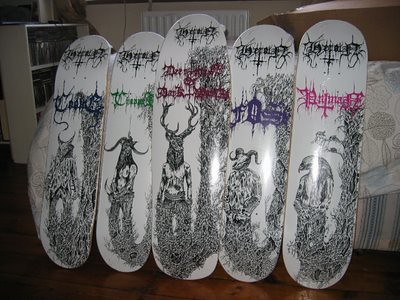The photo appears to be taken in a bedroom or living room, with what could be a couch or bed covered by a sheet or duvet in the background. Lined up side by side on the surface are five snowboard decks, each adorned with intricate, black-and-white designs. These designs depict humanoid figures with various animal heads, giving them a tribal tattoo-like appearance. The boards are differentiated by colored lettering, indicating they might be from the same brand.

Starting from the left, the first snowboard features dark blue lettering and depicts a muscular humanoid figure with what appears to be a skull and goat horns, giving it a demonic appearance. The second board, with green lettering, showcases a humanoid body topped with a satyr-like head, complete with curling horns. In the center, the third board has red lettering and displays a figure with a deer head and prominent antlers. The fourth snowboard, distinguished by purple lettering, shows a humanoid figure with an animal head that has a thin face and two horns, possibly resembling an anteater or similar creature. Finally, the snowboard on the far right has pink lettering and features a humanoid body with an eagle's head, complete with sharp beak and striking eyes.